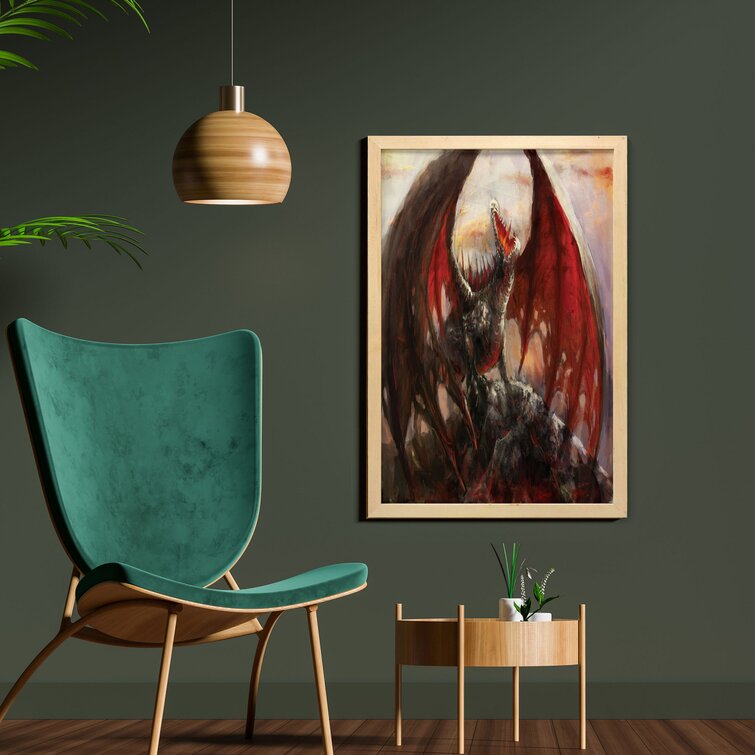The image depicts a living room or seating area, most likely created using computer graphics. Dominating the backdrop is an olive green or gray wall with a framed painting of a roaring dragon, featuring dark tones, red wings, and a light brown border. On the left side, there's a vintage green suede chair with wooden arms and legs. Above the chair hangs a dome-shaped brown lamp from the ceiling. A small light wooden table sits in the center, slightly to the right, adorned with two potted plants. The overall scene is detailed with wooden elements and touches of green, red, and brown, giving it a cozy and fantastical ambiance.